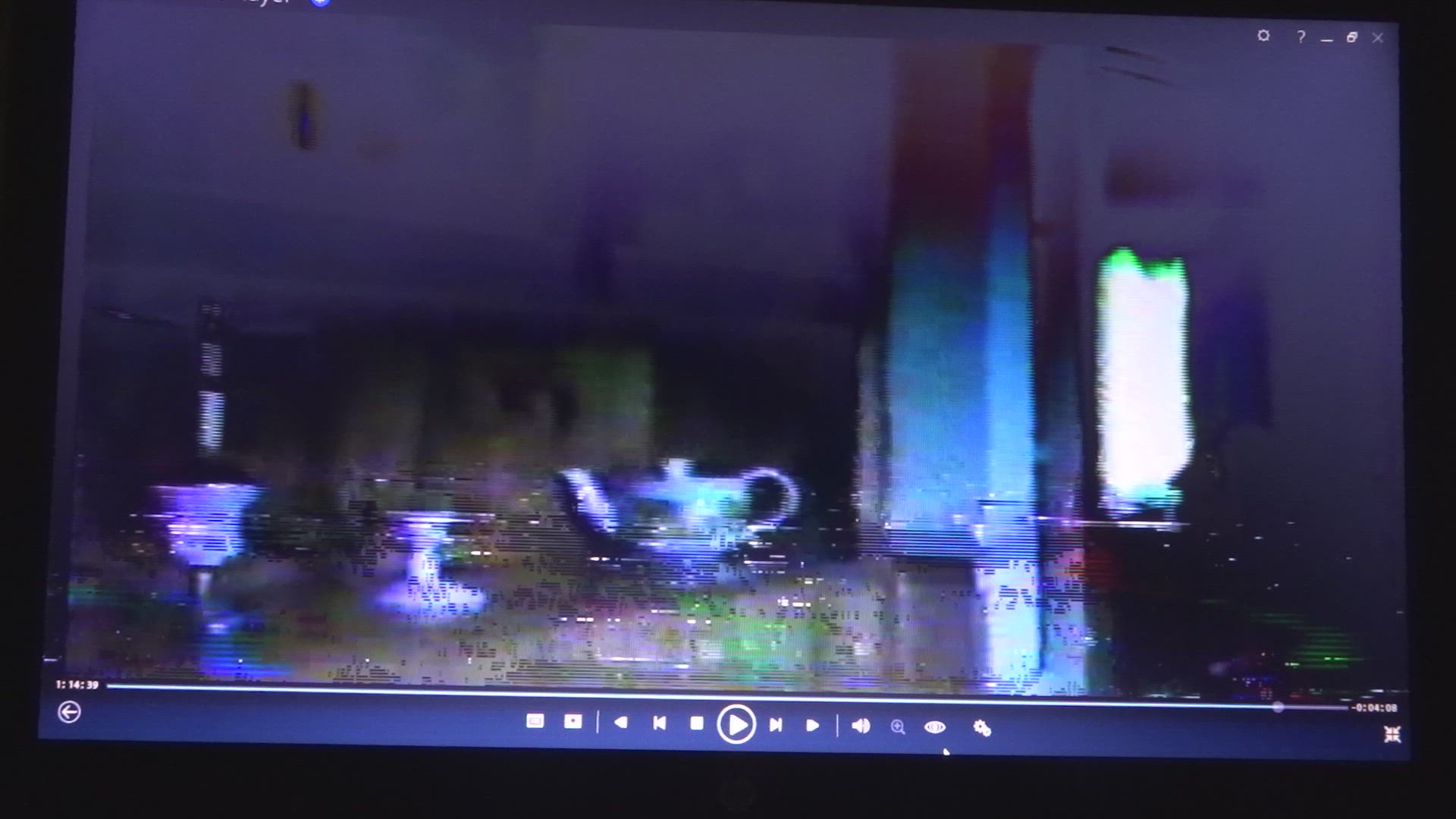The photograph depicts a computer screen with a prominent black trim around the edges. At the bottom of the screen, there is a dark blue taskbar filled with various icons, suggesting it might be a Windows operating system. A play button, timestamped at an hour and fourteen minutes and thirty-nine seconds, is clearly visible, indicating a video in progress. The image on the screen is quite blurred and pixelated, making it difficult to discern precise details.

However, in the central portion of the screen, there is a visible blue teapot, and on the left side, there's a silhouette resembling a goblet or a cup with a stem. The overall color scheme of the picture on the screen is a mix of light blue and dark blue, with the background featuring shades of purple. At the very top right, there are small white textual elements, perhaps indicating window controls like minimize, maximize, or close.

Additionally, scattered white lines across the image give it a static-like appearance, reminiscent of old, degraded video tapes. While the specific contents of the video or image are difficult to identify, the visual artifacts and overall blurriness contribute to a nostalgic, somewhat chaotic aesthetic.